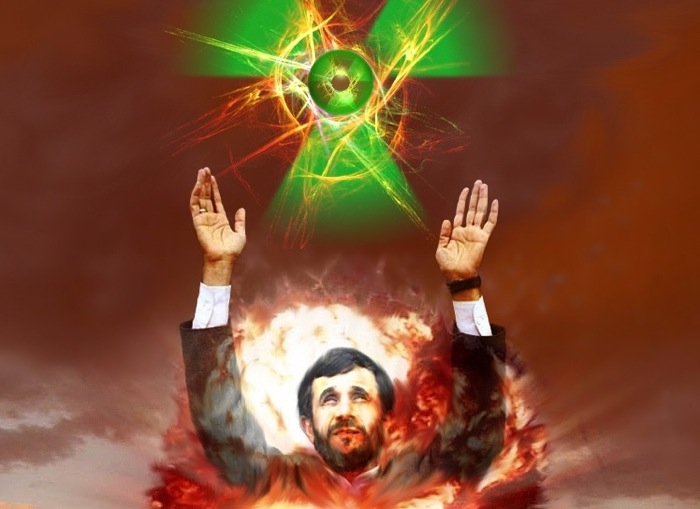In this vividly detailed image, a man with black hair and a black mustache, identified as the leader of Iran, stands prominently in the bottom middle of the frame. He is dressed in a dark blazer with white collar and cuffs, with his arms raised towards the sky. Surrounding him is a chaotic swirl of reddish-brown and white colors resembling flames and smoke, suggestive of a nuclear explosion or an intense firestorm. Above the man's head floats a mysterious green object with three branching arms, circled by yellow and reddish streaks, giving the impression of a glowing, windmill-like symbol. A white flash illuminates behind his head, enhancing the dramatic and apocalyptic atmosphere of the scene.